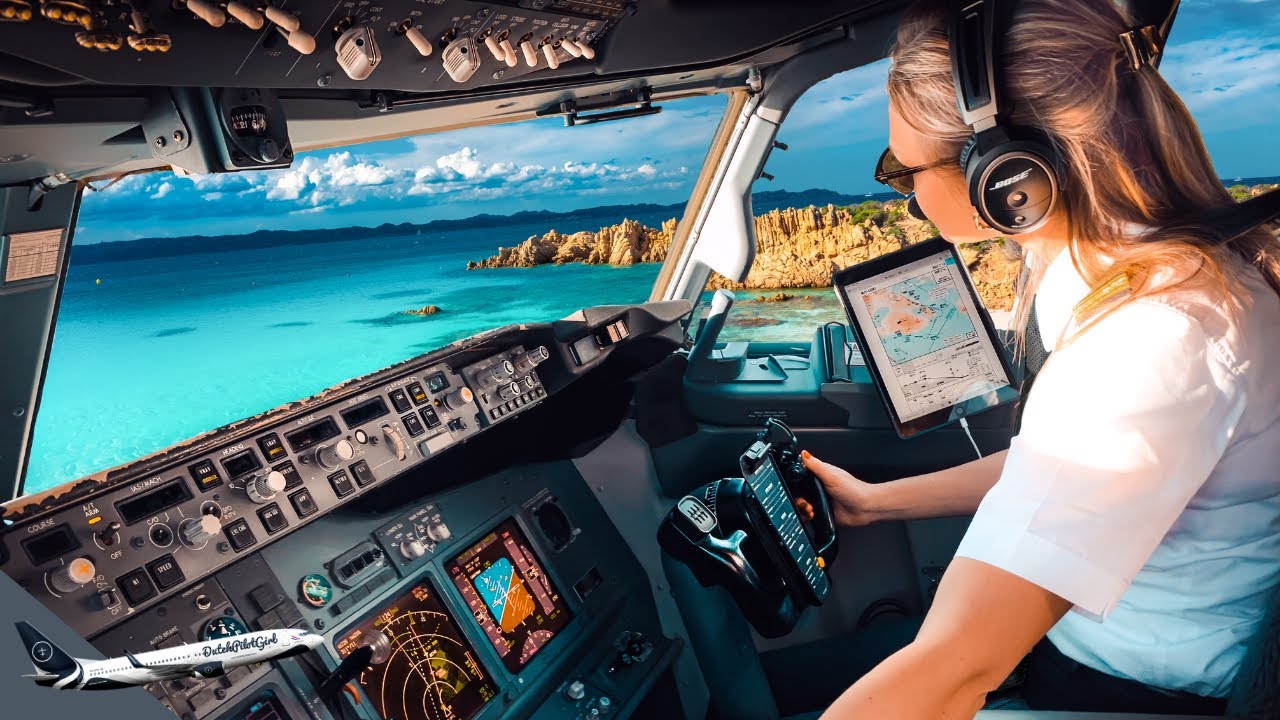In this image, a woman is piloting a modern aircraft and can be seen sitting comfortably in the cockpit. The woman, who has shoulder-length brown wavy hair, is wearing a short-sleeved white button-up dress shirt, a blackish tie, Bose earphones, and sunglasses. To her right is an iPad displaying flight controls, surrounded by a multitude of screens, buttons, switches, and toggles. Out the large cockpit windows, she gazes at the breathtaking seascape below.

The view showcases a stunning turquoise sea with both light and dark blue hues, which appears calm with minimal waves. Along the shoreline, there are tan cliffs and low-lying rocky formations, possibly indicating a Mediterranean or Caribbean setting. In the background, there are hills or mountains adorned with sparse vegetation, under a generally sunny sky dotted with scattered clouds. Off in the distance, ominous thunderstorm-like clouds loom, adding a dramatic element to the scene.

In the bottom left corner of the image, a large commercial airplane, likely a Boeing 737-800, is visible. The plane is predominantly white with blue accents on its engines, underbelly, and tail fin, although the writing on its side is indiscernible. The overall picture exudes a blend of serene and captivating elements, capturing a moment of tranquil beauty from the cockpit.